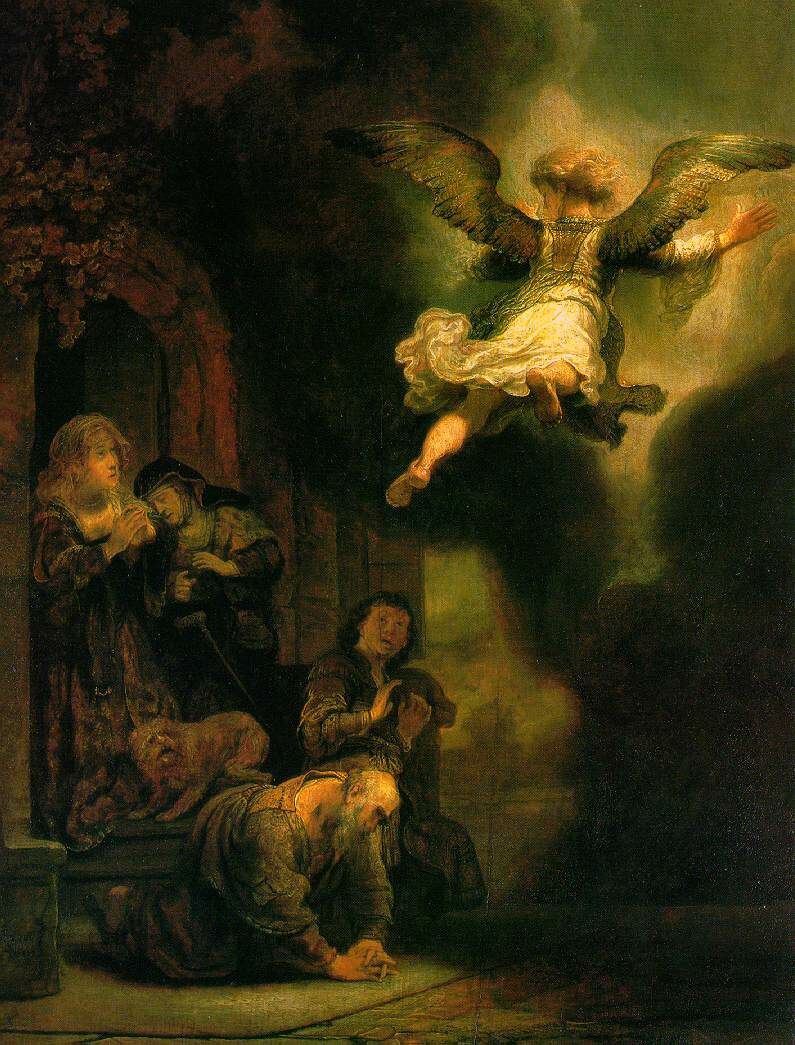In this detailed fine art oil painting, set in what appears to be a dark and moody medieval or Renaissance scene, an ethereal angel with flowing golden-yellow and green wings ascends towards the ceiling, radiating light. The angel, a young girl in a flowing white dress, is barefoot and looks down upon the figures below with outstretched arms. The scene is dominated by deep greens, blacks, and browns, adding to its somber tone.

On the left side, we see a group of four individuals and a small brown dog amidst an archway covered in flowers that frames the scene. The people are positioned as if in a moment of divine encounter. Foremost is a man on his knees, a gray-bearded figure with an open collar, who clasps his hands in prayer and gazes upward. Behind him stands a woman with loose, reddish-brown hair, also in prayer, her eyes fixed on the angel above. Another woman, veiled in black with a melancholy expression, stands slightly behind, her hands clasped together as she looks downward. A small brown dog sits between the women, looking up at the angel with a curious expression. 

In the background, another archway reveals the presence of a man with a bald head and an open collar, surveying the scene with a mix of reverence and shock. His anxious posture, with hands raised as if guarding himself, encapsulates the chaos and wonder evoked by the angelic visitation. The room's dark green tones and the figures' rich, period-appropriate attire further enhance the painting's historical and mystical ambiance.